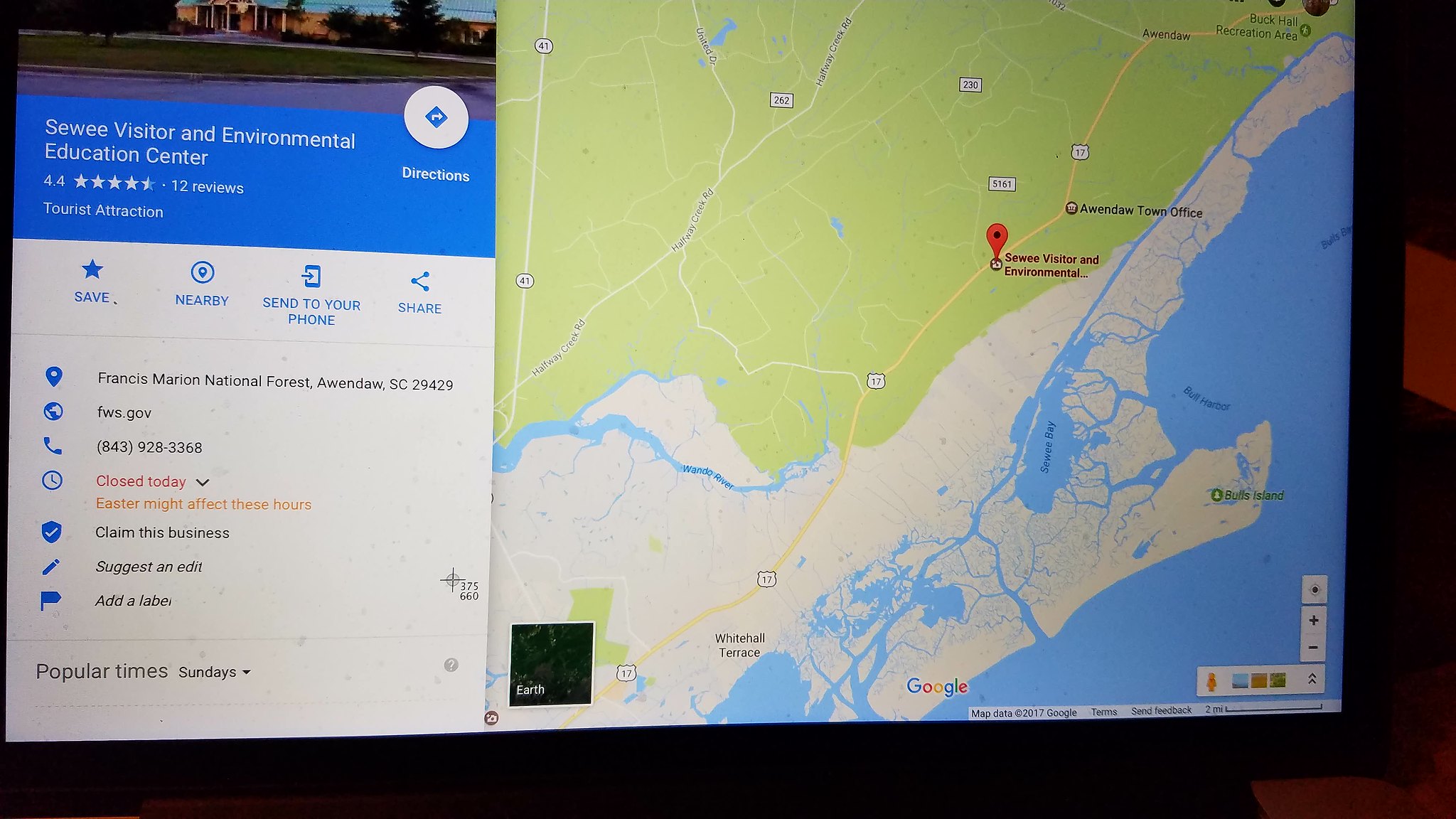This image is a screen capture of a computer screen displaying a map application focused on the Seawee Visitor and Environmental Education Center. The center, considered a tourist attraction, has a rating of 4.4 from 12 reviews on Google. On the left side of the screen, there are directions to reach the center, located in Francis Marion National Park, Arwen Door, SC 29429. The page also includes a website link to fws.gov, a phone number, and notes that the center is closed today. Options to claim the business, suggest an edit, and add a tab are also visible. To the right, a coastal map shows the location in detail with a highway system highlighted. The map uses blue to indicate the ocean, white for landmass, and green overlays potentially marking county or state boundaries.